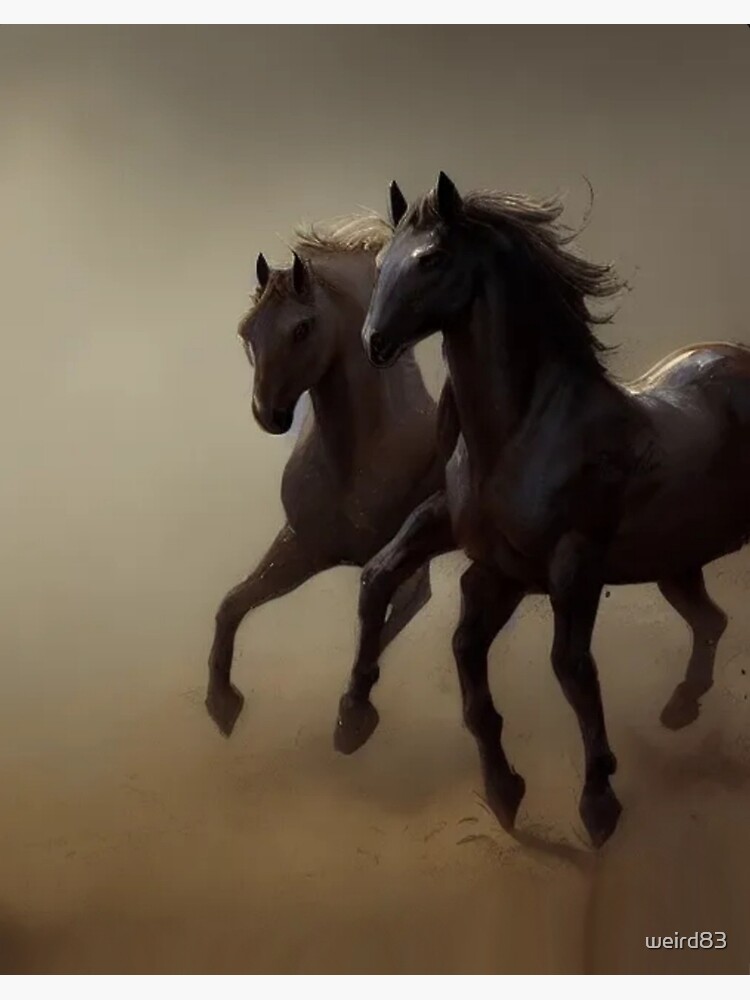The image is a digitized or possibly watercolor painting featuring two horses running against a grayish, dust storm-like backdrop that transitions into a dirty, tannish ground. Central to the composition are two horses: the one on the left is smaller, brown, and has all its legs raised mid-jump, creating a sense of dynamic motion. The horse on the right is larger, darker, and appears to be a mix of black and brown hues. Its front legs are on the ground, but the rear legs are not visible in the image, possibly obscured by the other horse. Both horses have their manes flowing dramatically, amplifying the sense of speed and movement. Intricate details are noticeable in the design accents on the horses and the texture of the canvas, blending seamlessly into the overall story of the artwork. At the bottom right corner, the phrase "Weird 83" is inscribed in white text.